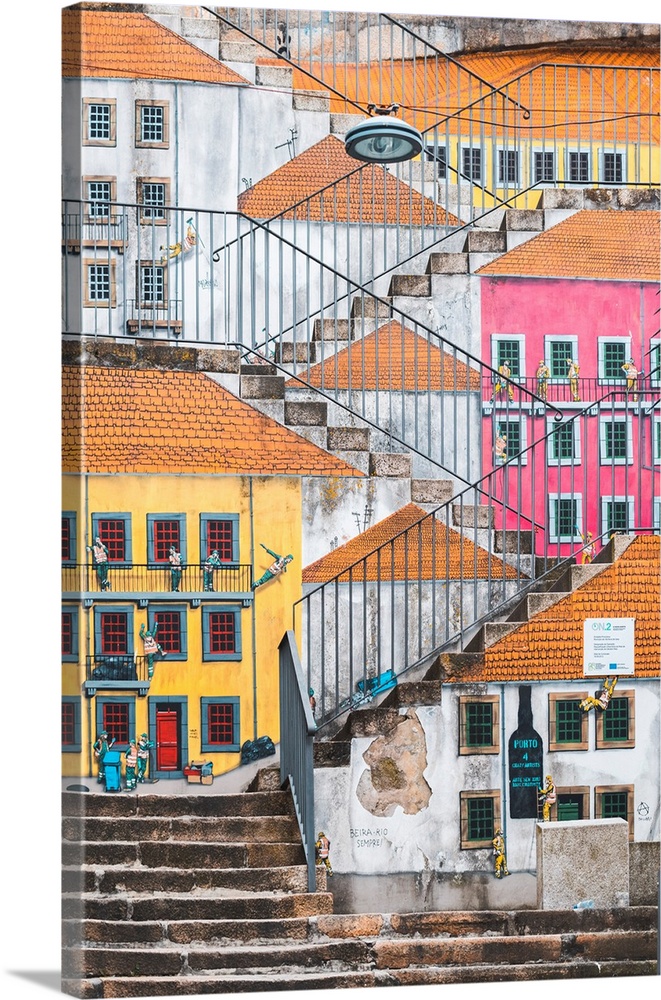The image depicts a detailed painting of several interconnected, multi-colored buildings arranged on varying flights of stairs. The buildings, which appear European in style, include colors such as yellow, pink, white, and tan, and are depicted with brown shingled, slanted roofs. The staircases zigzag through the painting, connecting the different buildings, creating a layered effect. On the bottom floor, there is a white building with visible cracks, and adjacent to it is a yellow building where flat, red-outlined figures of people are seen next to the windows. Higher up the stairs is a pink building with similar figures, and further up to the right is another white building with a single figure. The painting is displayed on a thick canvas that casts a shadow, indicating it stands freestanding in a white room. Additionally, a black wine bottle is painted on one of the walls towards the lower part of the composition.